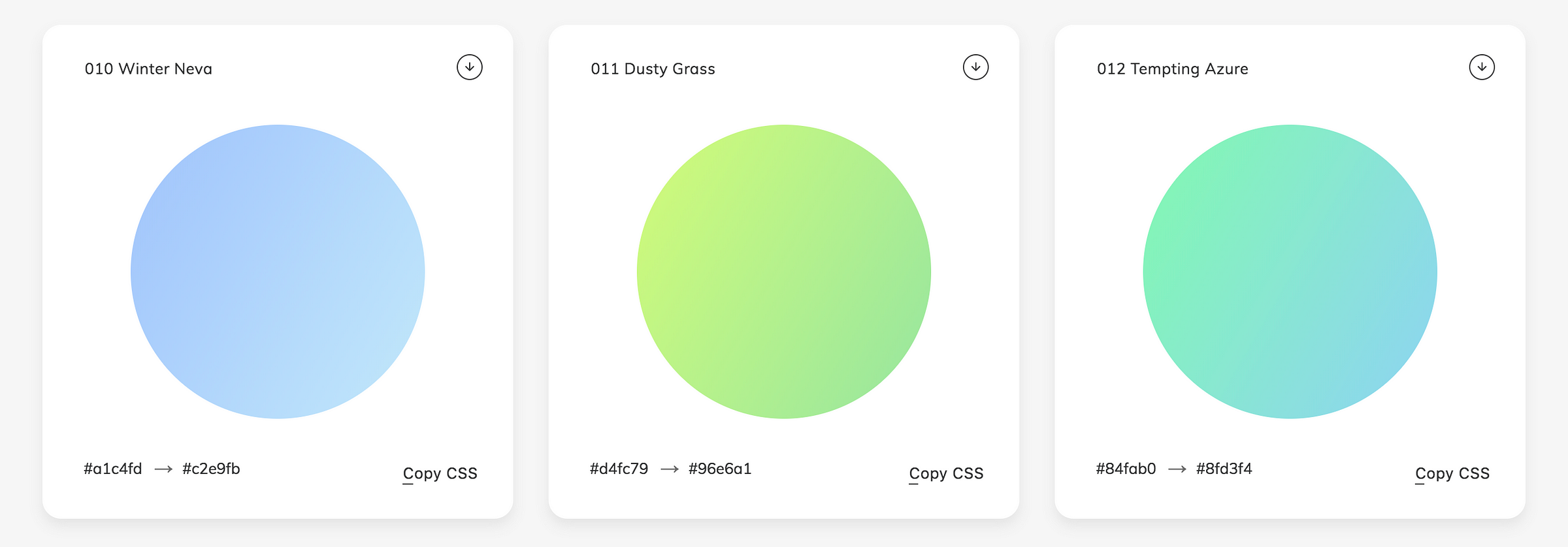The image depicts a set of three circular color swatches, each featuring a distinct gradient and labeled as if they were paint samples. These swatches are likely digital representations, possibly showcasing web color options.

1. The leftmost circle is labeled "010 Winter Neva." This swatch displays a delicate pastel baby blue gradient, evoking a sense of cool serenity. Above this circle, an arrow within a circle points downward, indicating additional options or actions.
   
2. Alongside "Winter Neva," a horizontal arrangement displays a code with an arrow pointing right, leading to another code, suggesting a transition or conversion between color codes. Below this arrangement, the option "Copy CSS" is available, allowing users to easily copy the cascading style sheet (CSS) code for the color.

3. The second circle in the sequence is titled "011 Dusty Grass," presenting a gradient of lime green. This color suggests freshness and vibrancy, reminiscent of spring grass.

4. The final circle is named "012 Tempting Azure," featuring a gradient blending lime and aquamarine hues, creating a dynamic yet harmonious palette.

Overall, the image appears to be a visual sample of different gradient color options, possibly designed for web or graphic design applications, each with convenient tools for code transition and CSS copying.